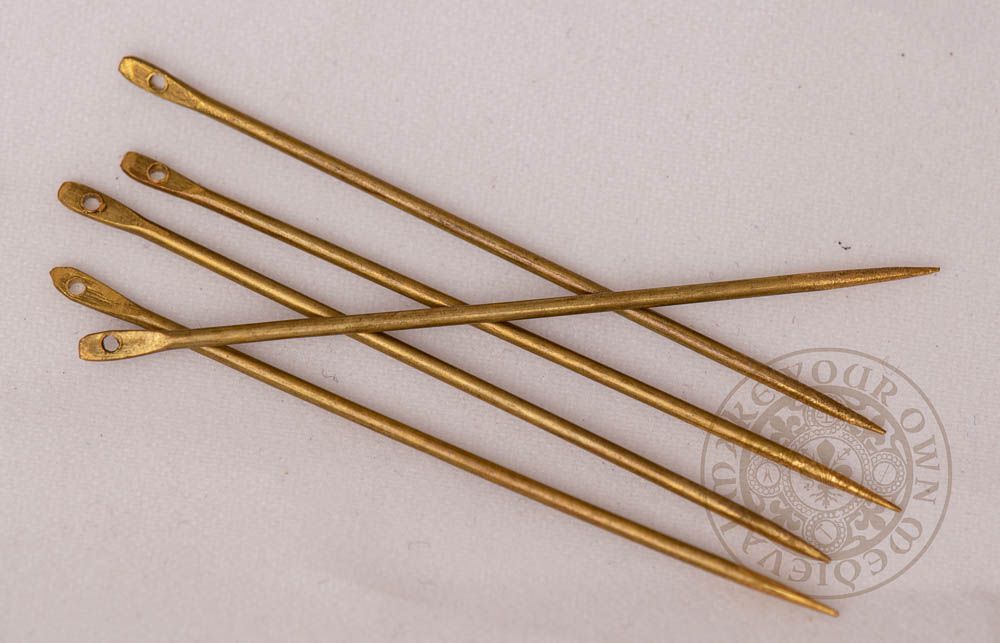The image depicts five antique sewing needles, arranged diagonally on a plain cream-colored paper. The needles display a copperish bronze hue, with signs of significant age, including tarnish and almost black spots. Measuring larger and thicker than standard modern needles, these decorative implements feature a pointed tip at one end and a flattened end with a small hole suitable for threading string. Four needles are aligned in a row, while the fifth needle is placed across the top of the others. In the bottom right corner, there is a partially legible emblem that reads, "Make Your Own Medieval Ware," accompanied by a distinctive design that resembles a medieval or potentially foreign symbol.